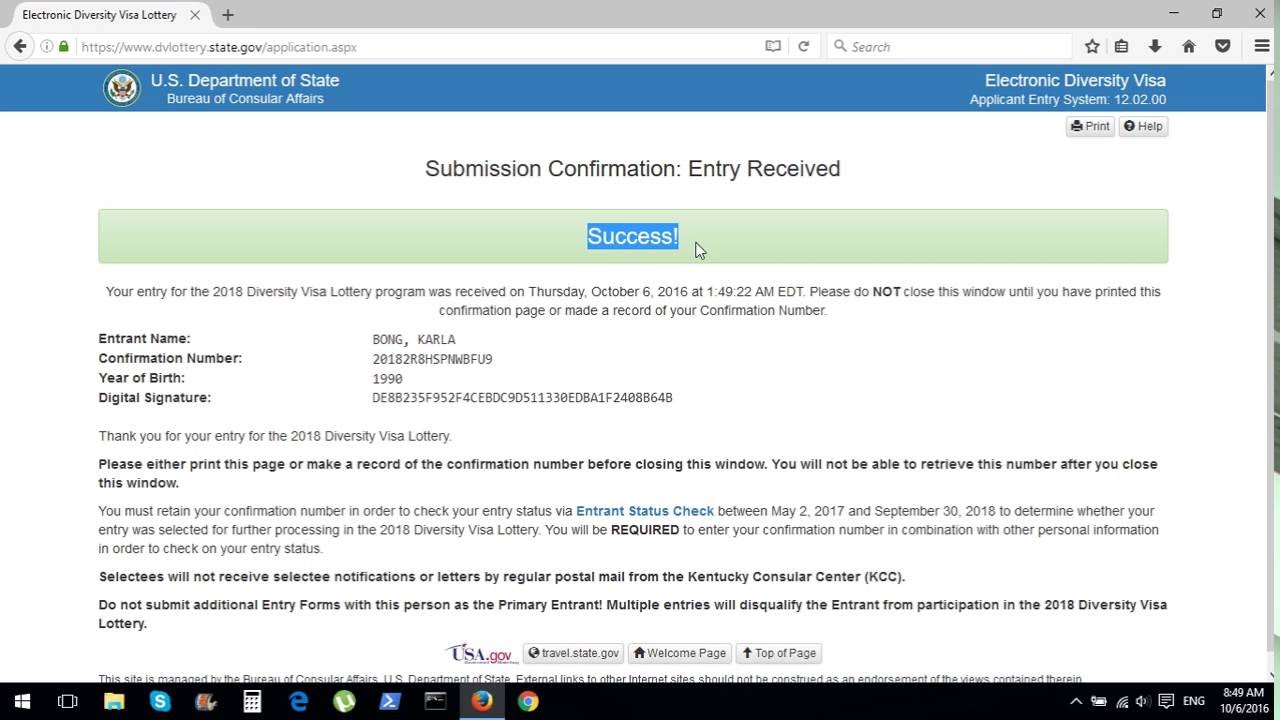The image is a detailed screenshot of a webpage, bordered on the top and bottom by the browser interface and computer taskbar, respectively. At the very top left of the screenshot, there is an open tab. Extending across the top is a dark gray browser toolbar, which includes a minimize button, a new tab button, and a close button located at the top right.

Directly beneath this gray toolbar is a white URL box on the left and a search box on the right. Below these elements, the main content of the webpage begins. The upper portion of the webpage features a large blue rectangle background. On the far left of this blue rectangle is the logo for the U.S. Department of State, accompanied by the text "U.S. Department of State Bureau of Consumer Affairs" in white.

The remainder of the webpage has a white background. Prominently displayed at the top is a title in black text that reads "Submission Confirmation Entry Received." Directly below this title, the word "Success" is highlighted within a blue rectangle with white text. Beneath this, there is a block of very small black text explaining the submission details.

At the very bottom of the screenshot, the black taskbar of the computer is visible. This taskbar features various icons for websites and programs. The background of the entire image is white, emphasizing the contrast between the webpage content and the browser and taskbar interfaces.